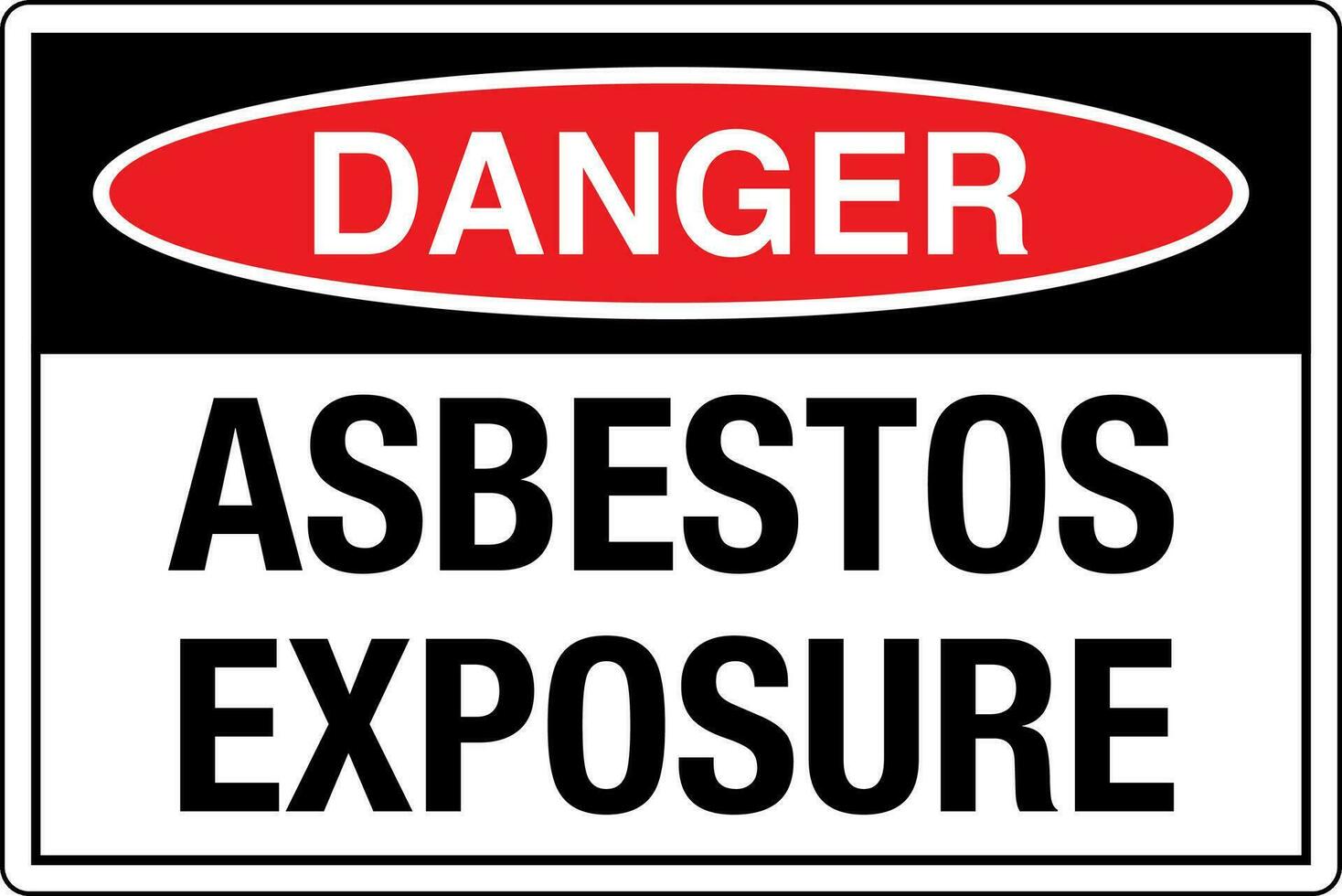This image displays a rectangular warning sign designed with a blend of black, red, and white colors. The sign features a thin black border, followed by a slightly thicker black border encapsulating the entire sign. At the very top, there is a black band. Below it, within a white-bordered red oval, bold white text spells out "DANGER." The lower two-thirds of the sign, set against a white background, contains bold black text stating "ASBESTOS EXPOSURE." This sign appears to be digitally created using graphic software, seemingly intended for print rather than as a physical sign. The purpose of the sign is to alert individuals to potential asbestos hazards, prompting the use of appropriate personal protective equipment (PPE) such as masks to prevent the inhalation of dangerous asbestos fibers.